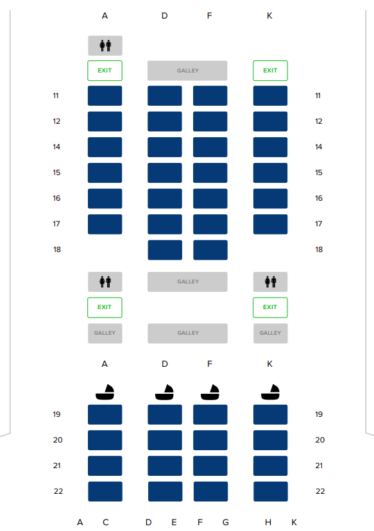This is a detailed overhead screenshot depicting the seating arrangement of a plane's midsection. At the top of the image, the letters "AD," "F," and "K" are prominently displayed, accompanied by male and female symbols, indicating the presence of restrooms. Flanked by two exit signs, the central "Galley" area is highlighted in gray. 

Following this, there are four rows of seats from 11 to 18, aligned in a 3-3-3 configuration, with aisles separating the seats. Notably, row 18 lacks window-side seating. Below this, another "Galley" area is positioned in the center, bordered by two more restrooms and exit signs.

Further down, the seating arrangement continues with rows 19 and 20, where small icons, depicting bassinets for infants, can be seen. The image concludes with the row denotations "AC," "DEFG," and "HK" at the bottom. Light gray lines running along the sides represent the fuselage walls. This illustration captures a comprehensive view of the aircraft's middle section, detailing the spatial configuration and essential amenities.